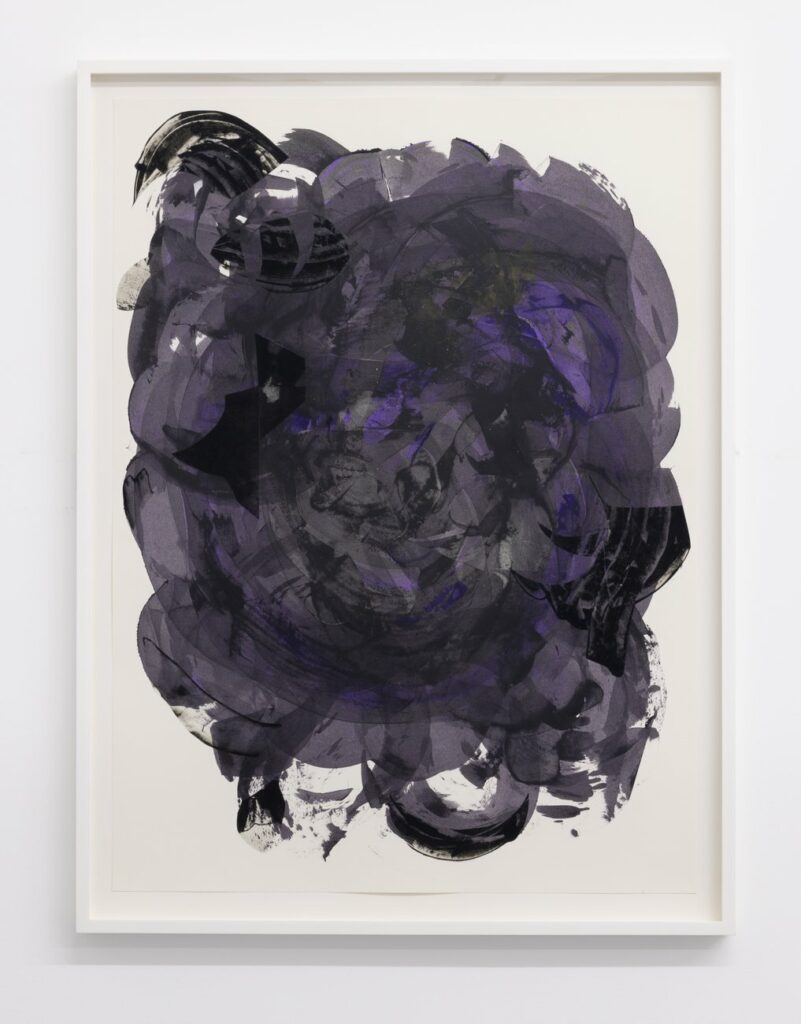This is a photograph in portrait mode of a modern, abstract painting framed in white and hung on a white wall. The painting resides within a pure white frame, while the canvas or paper it is on has a very light cream or off-white background. The artwork itself is a dynamic and chaotic mix of black, gray, and various shades of purple, featuring numerous swirling and wave-like paint strokes. At the top left-hand corner, there is a distinct black wave that juts out and then shoots downward. The bottom of the painting is underlined by a curved wave of black, which anchors the swirling mass above. The overall effect is that of an intense, swirling, almost angry chaotic mass, as if someone took a paintbrush and fervently swished and swirled the colors together in a circular and wave-like fashion.